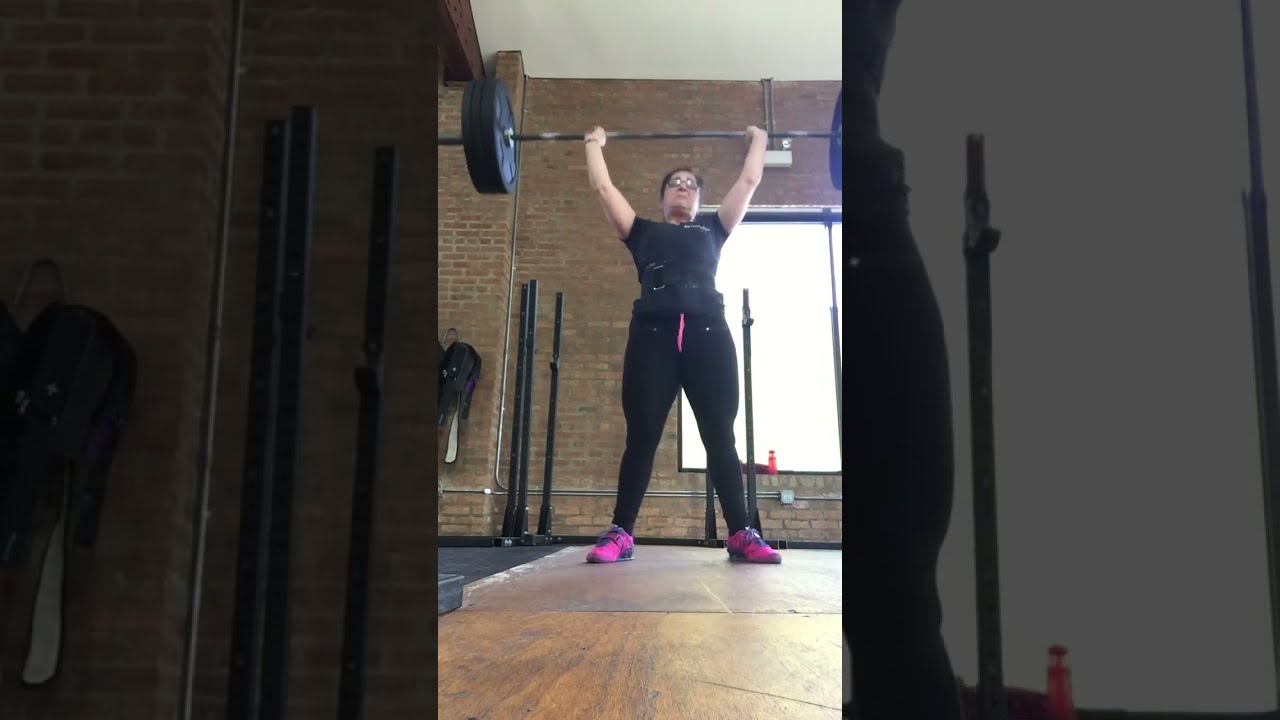In the image, a woman is captured in the midst of an intense workout session, lifting a heavy barbell laden with black round weight plates above her head. She has dark brown hair and is donning black-rimmed glasses, indicating her Caucasian ancestry. She is dressed in a black compression t-shirt and black leggings, accentuated by pink drawstrings, and completed with pink and blue (or purple) sneakers. To support her heavy lifting, she wears a black weightlifting belt around her waist. The setting is a gym with a rubber mat over a wooden floor, brick walls in the background, and a window letting in white light. Additional details include visible conduit pipes, backpacks or similar equipment hanging on the wall, and a red sports drink placed on the windowsill. The woman's muscular legs and overall physique underscore her dedication to fitness, although her facial expression suggests she might be feeling apprehensive or challenged by the weight she's lifting.